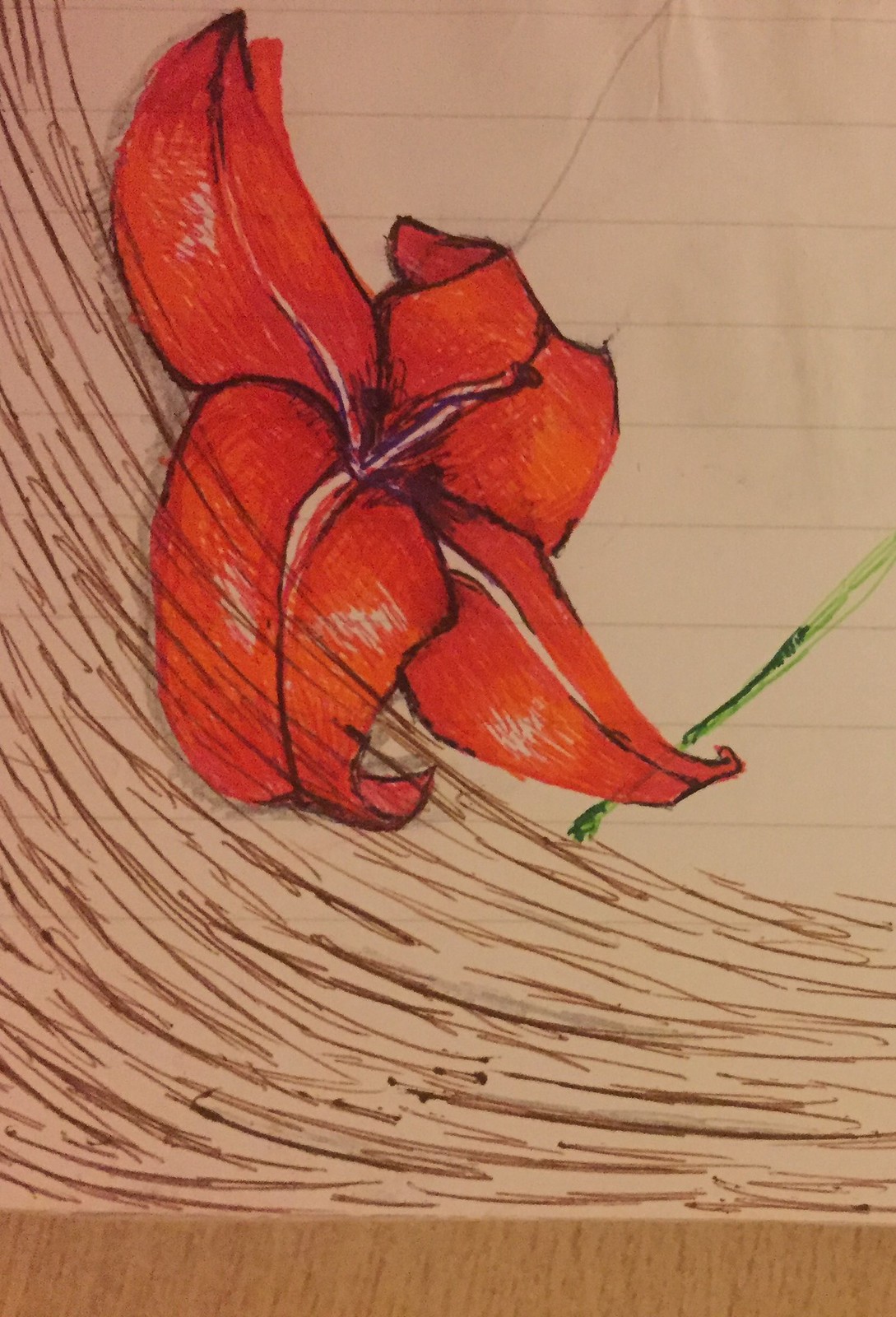The image showcases an illustration of a red flower on lined notebook paper. The flower features at least four red, intricately detailed petals, each with a slight variance in hue, displaying streaks of purple ink that add depth and texture. The flower’s center reveals a complex, stringy area and a tubular structure, providing a focal point of interest. To the right of the flower, a green stem-like structure can be observed, positioned off-center and adding a touch of organic realism. Below the flower, towards the bottom left side of the image, there are numerous hatched black lines, possibly created with pencil or pen, forming a curved pattern that enhances the overall composition.